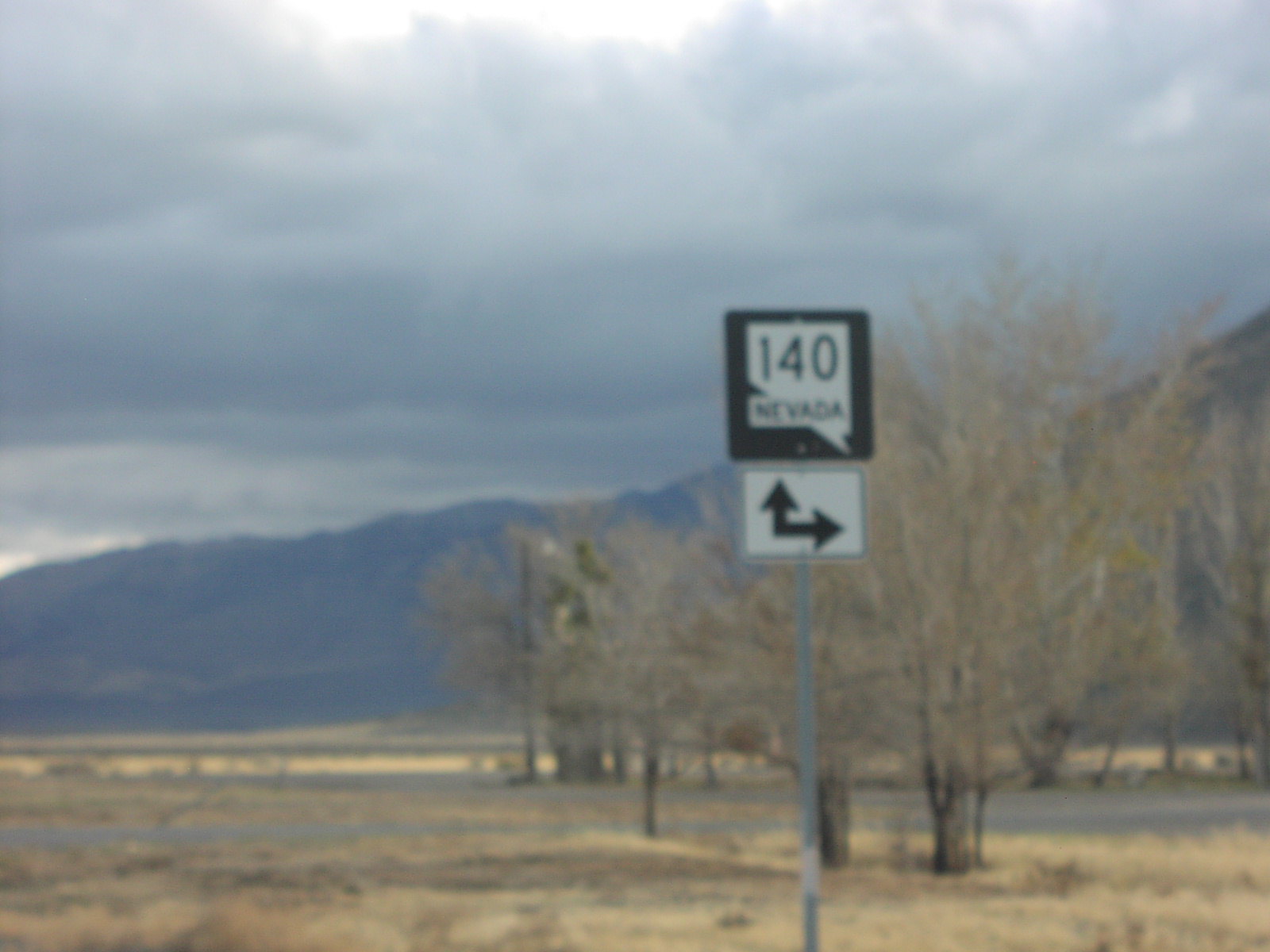This image captures a rural Nevada landscape through a slightly blurry photo, likely taken from a moving vehicle. Dominating the scene is a road sign positioned about one-third of the way from the right. The sign features a metal pole that extends halfway up the image before it disappears behind a dense cluster of lush, green, and brown trees. On the sign, a thick black arrow points upward, with another extending to the right, both set against a white background. Above this, a black square displays the number "140" in white, set within the sharply angular outline of the state of Nevada, also labeled "Nevada."

Below the sign, the ground is a mix of dry, beige grass and patches of green, suggesting late autumn or early winter. The background is filled with more trees, fewer in number and with sparse foliage, hinting at the season. Beyond the trees, a dark greenish mountain range stretches across the middle of the image, initially level before rising at a sharp angle towards the right.

The sky above is thick with dark, heavy clouds, casting a gloomy atmosphere over the scene. However, there is a faint glow where the sun attempts to break through at the very top of the photo, contributing a subtle contrast to the overall grey and overcast mood. The landscape beneath, with its open, slightly desolate feel, emphasizes the remote and serene nature of this Nevadan countryside.